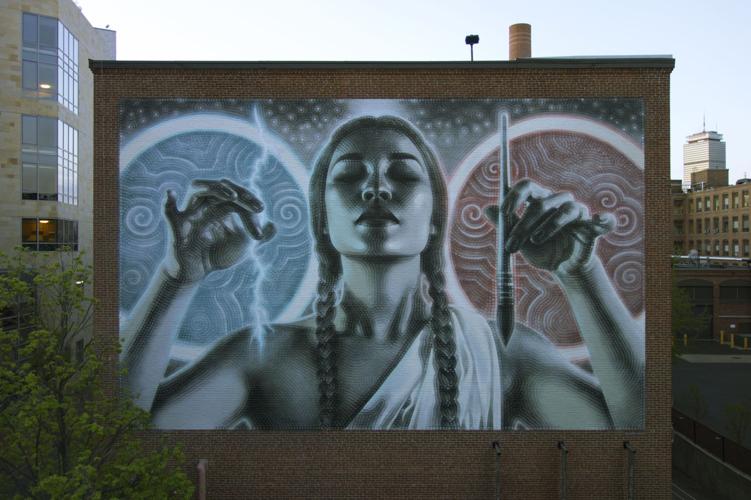The photograph captures an outdoor scene dominated by a cityscape, with a large, squared, brown brick building as the focal point. The background features a light blue sky. Painted on the facade of this building is a striking and somewhat psychedelic mural of a young woman, approximately 18 years old, depicted in black and white. The woman, framed by two glowing circles—one with a white outline and a blue center on her left, and the other with a white outline and a maroon center on her right—exudes an ethereal presence.

She stands with her head slightly tilted back, eyes closed, and extends her arms forward with a notable grace. Her hands hold symbolic items: a paintbrush pointing downward in her left hand and what appears to be a white lightning bolt in her right hand. She is adorned in a classic white toga over her left arm and shoulder, and her long hair is styled in two braids that cascade down the sides of her face and over her chest. Surrounding the mural, the city buildings emphasize the mural's grandeur and its apparent role in promoting art within the urban environment. Despite the muted colors, the image leaves a lasting impression with its dramatic and captivating artistry.